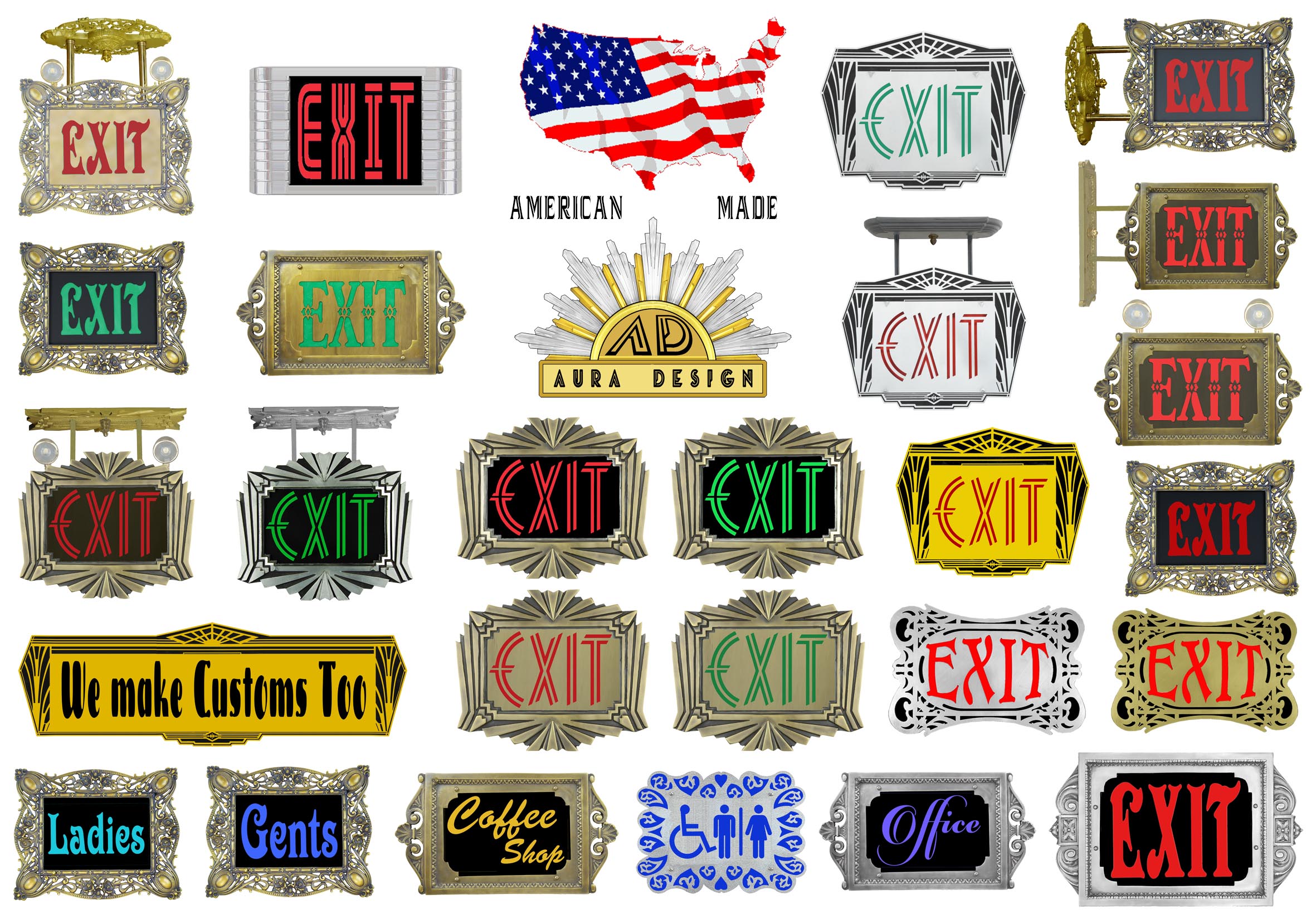The image showcases an extensive collection of about 40 distinct exit signs, intricately designed to vary in color, font, and shape—from square to circular forms. Most of these signs prominently display the word "exit" in vibrant colors like red and green, framed with styles ranging from simple to ornate. Positioned centrally, the text "Aura Design" with a sun logo and the initials "AD" is clearly visible, indicating the designer's brand. Prominent above this logo, the phrase "American Made" is displayed over a United States silhouette adorned with the American flag. Scattered amongst the exit signs are a few other signs for various facilities such as bathrooms (including an ADA-compliant symbol), an office, and a coffee shop. Additionally, a note in the corner mentions that custom designs are available, highlighting the company’s versatility. This image essentially functions as an advertisement for Aura Design's creative and diverse sign-making capabilities.